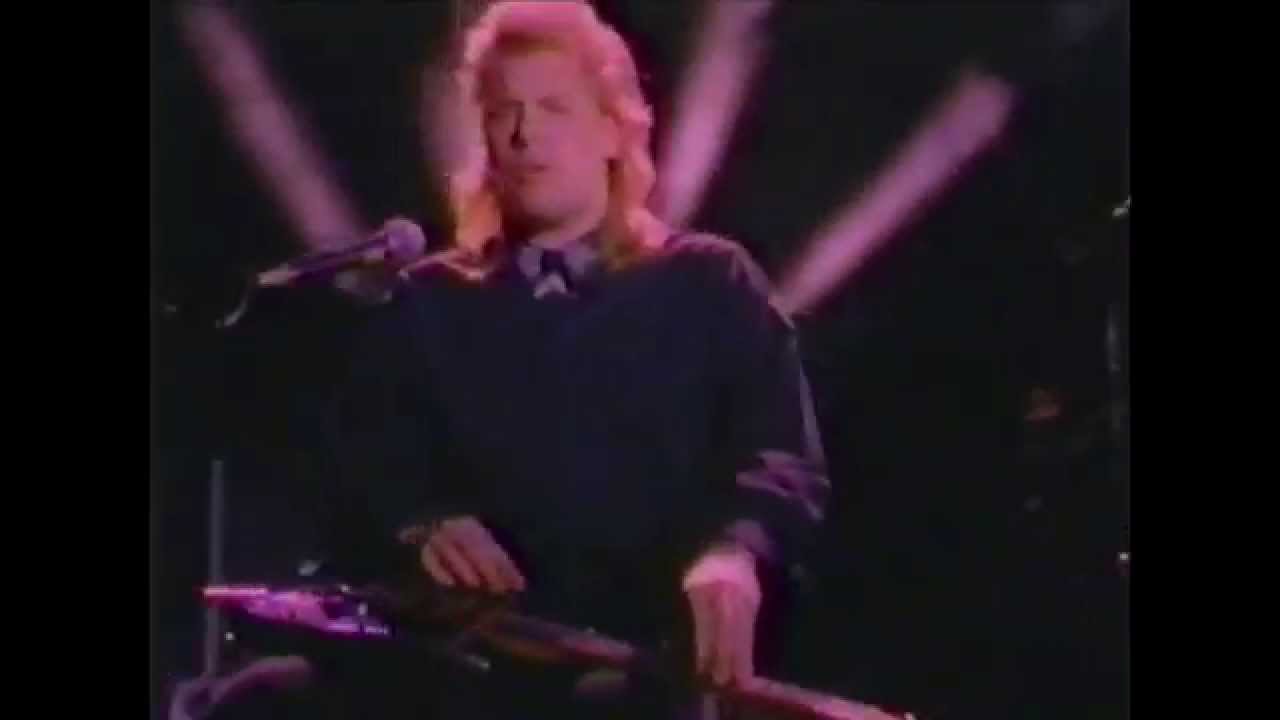The image captures a nostalgic scene evocative of an 80s music video. Central to the frame is a man with long, gold-blonde hair, styled into a mullet, suggestive of the era. He is simultaneously singing into a microphone situated on a mic stand and playing a keyboard, possibly with a guitar or another instrument resting on his lap. His attire includes a gray, button-up shirt, buttoned all the way to the top, under a V-neck sweater, paired with dark pants—complete with an 80s flair. Despite the blur, a black background accentuates the stage-like setting, accompanied by dramatic lighting: multiple purple spotlights cascade around him, enhancing the overall cool ambiance of the performance. The purple hues cast a soft glow on his figure, adding to the concert's vibrant aesthetic.